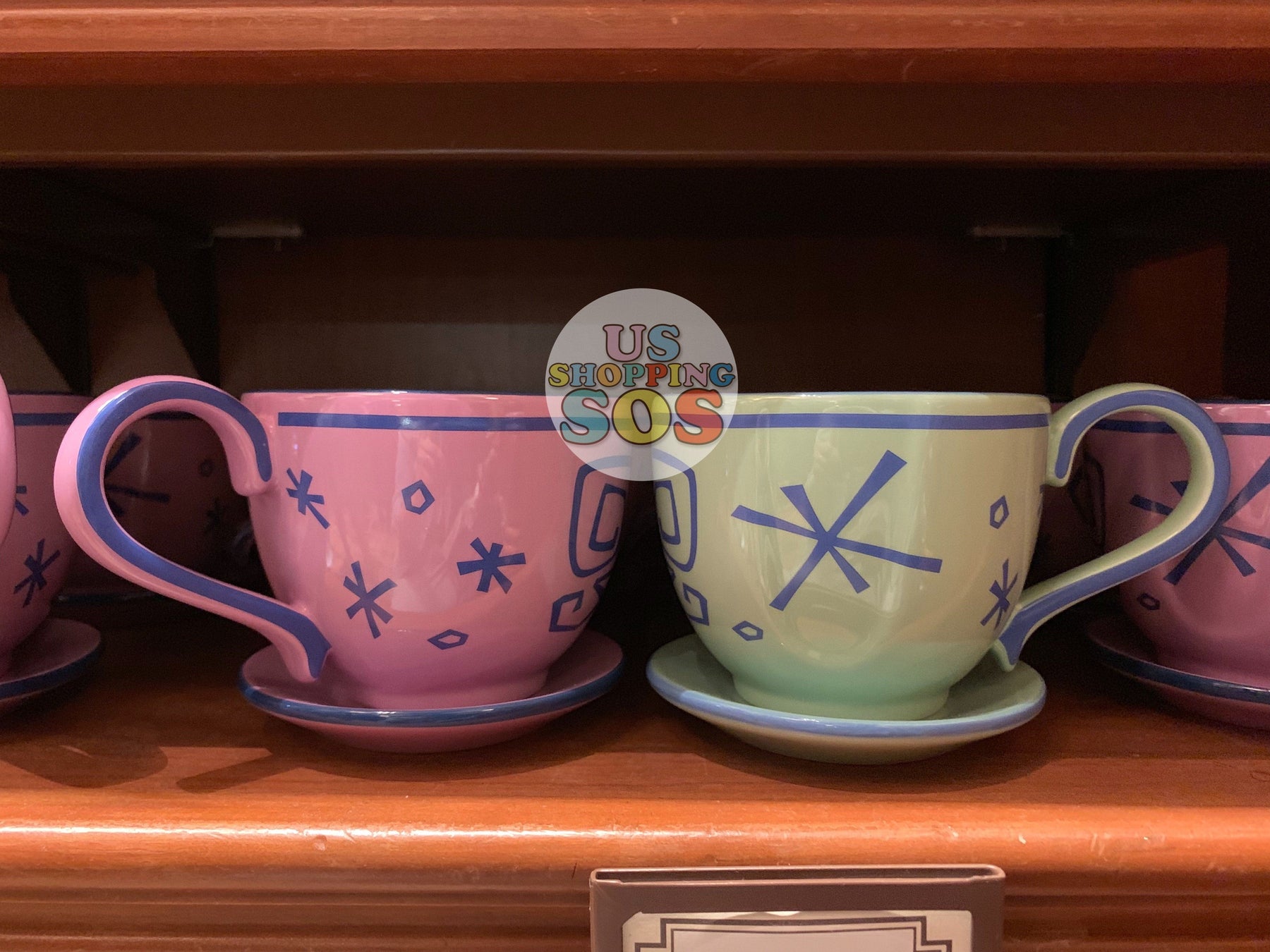The photograph depicts a collection of playful, stylized coffee mugs resting on a wooden shelf. In the center of the image, there are two prominent mugs: one in a light sage green with blue star asterisk-like designs and another in pink with similar blue detailing. Both mugs feature matching platters adorned with circles and asterisk patterns. Surrounding these central mugs are additional pink ones, making a total of four visible pink mugs. The mugs are part of a cohesive set with long, curvy handles and intricately detailed bases. Superimposed on the image is a slightly transparent white circle with colorful, multicolored text reading "U.S. Shopping S.O.S." The setting appears to be an open-shelf wooden cabinet, giving a casual and homey vibe to the scene.